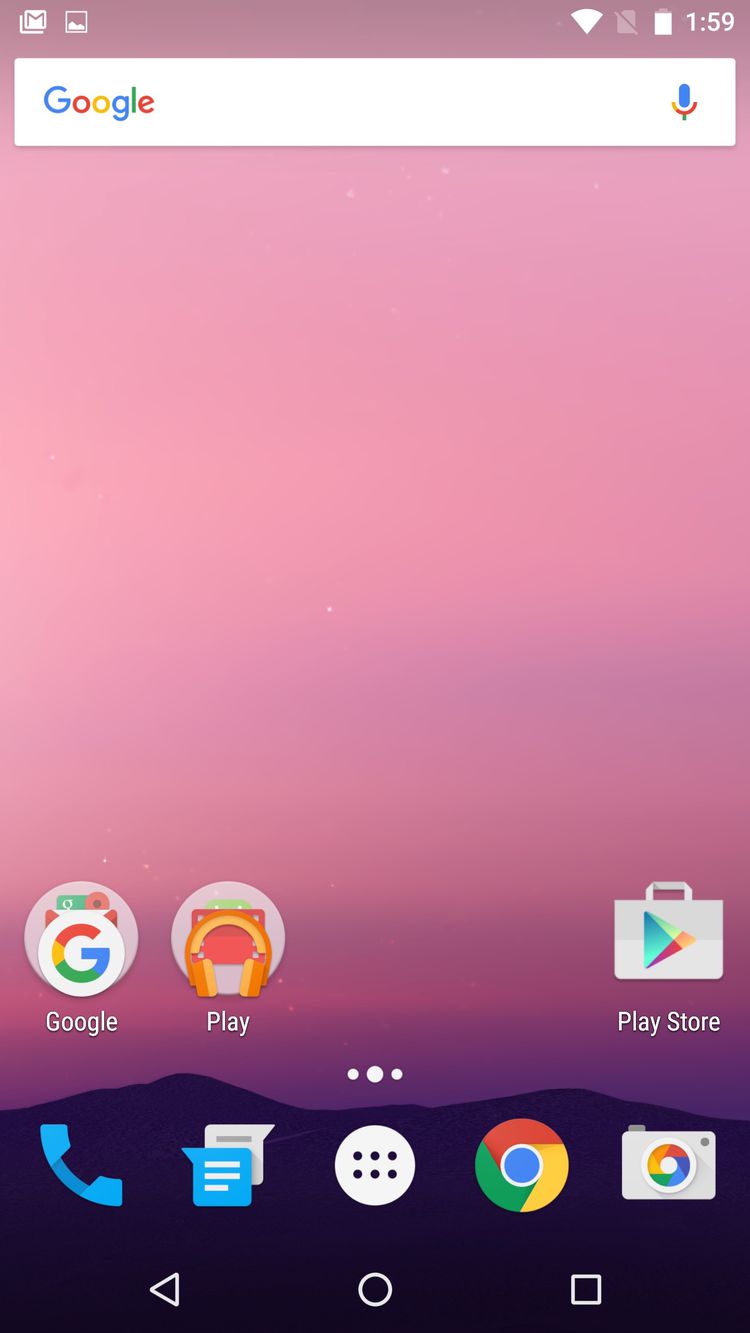This image captures a screenshot of a smartphone home screen set against a visually appealing background. The top portion features a search bar labeled "Google," conveniently equipped with a microphone icon within the bar itself. Surrounding the search bar, the time is prominently displayed as 1:59, with indicators showing a full battery and strong Wi-Fi signal.

The background image portrays a serene, gradient pink sky that transitions to a deeper hue as it approaches a dark purple silhouette of a mountain. The artwork presents a modern aesthetic with subtle details, like the gradual gradient darkening towards the mountainous horizon.

Below the sky, numerous app icons are neatly arranged. The visible icons include Google, Play, Play Store, Camera, Google Search, and a circle containing six dots, likely a launcher for more apps. Additionally, there are icons for messaging and making phone calls. Towards the bottom of the screen, navigation buttons for start, rewind, and stop are present, hinting at media or app control functionalities.

In the top left corner, additional icons serve as shortcuts to Gmail and Photos apps. Altogether, the screen features a total of eight app icons, blending functionality with an aesthetically pleasing and modern design.